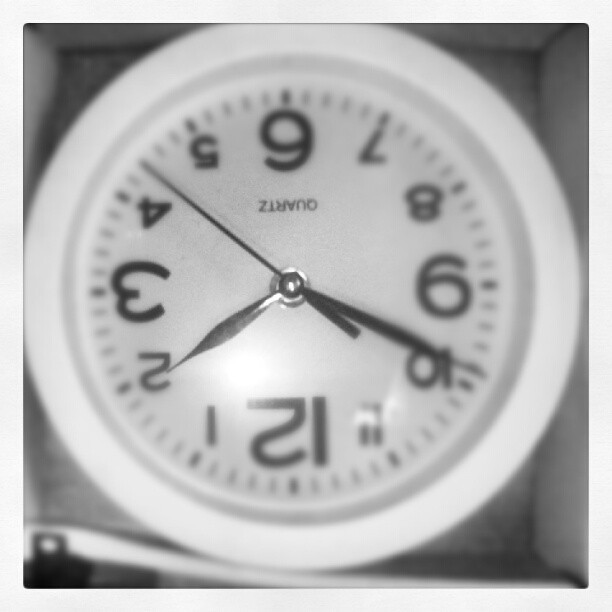This image features an upside-down clock, where the numeral 12 is positioned at the bottom and the 6 is at the top, indicating that the entire clock is inverted. Taken from a bird's-eye view, the photo is slightly distorted and somewhat blurry, yet the black-colored numerals are clear and easy to read. The clock has a very simple design, with both its face and surrounding frame colored in white. The scene hints at the clock being placed within a white box, adding to the minimalist theme. The image appears to be in black and white, as no other colors are visible. Near the bottom of the clock face, the word "quartz" is prominently displayed.